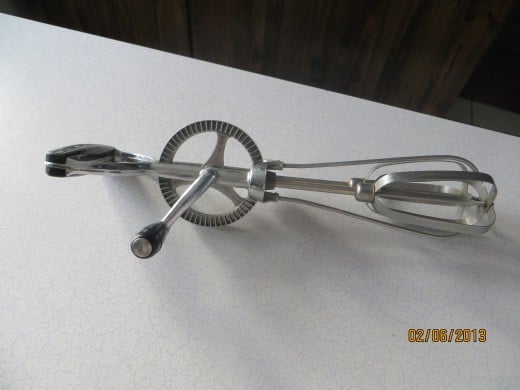The image depicts a vintage manual egg beater resting horizontally on a white countertop. The egg beater is composed primarily of shiny silver metal, featuring a small hand crank in the center with an attached black handle. The top handle, also black, provides a firm grip for the user. This utensil, measuring like a classic hand mixer, has two rotating beaters at the bottom that spin when the hand crank is turned. The background reveals wooden cabinetry and a tiled floor, with the date "02-06-2013" in yellow in the lower right corner, suggesting the photo was taken on February 6, 2013, likely with an old digital camera. The setting and the components of the image harken back to a simpler era of kitchen tools.